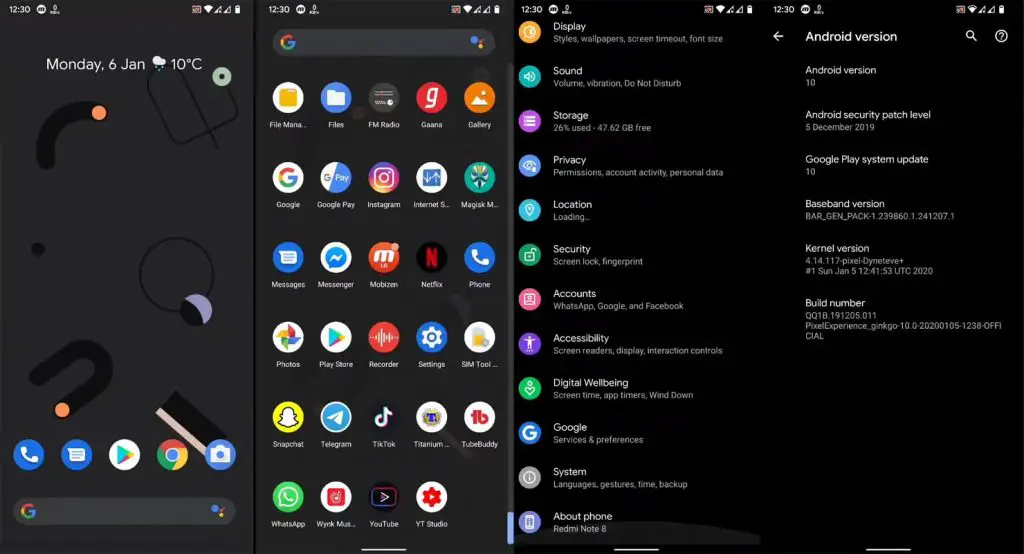The image depicts a black smartphone screen composed of four sequential screens. 

1. **First Screen:** 
   - The upper part displays the date and day: "Monday, January 6."
   - Current time: "12:30."
   - Weather information: A cloud with rain symbol accompanied by "10°C".
   - In the upper right corner are icons for cellular signal strength and Wi-Fi connectivity. 
   - Scattered across the screen are orange dots, whose function is unclear.
   - At the bottom, there are application icons for:
     - Phone 
     - Messages 
     - Google Play Store 
     - Google Search 
     - Camera

2. **Second Screen:**
   - Continues to display the time: "12:30."
   - At the top, there is a Google search bar.
   - The screen is densely populated with assorted app icons, inclusively:
     - File Management 
     - Files 
     - FM Radio 
     - Gallery 
     - Google 
     - Google Play Store 
     - Instagram 
     - Internet 
     - Messenger 
     - Messages 
     - Google Pay 
     - Netflix 
     - Phone 
     - SMS 
     - Digital Wellbeing Tools 

3. **Third and Fourth Screens:** 
   - Both screens predominantly feature navigations related to the device's settings. 
   - These likely include various sub-sections and options available within the settings menu on an Android operating system.

Overall, the series of screens offers a detailed glimpse into the smartphone's user interface, emphasizing both frequently used applications and critical settings accessible to the user.